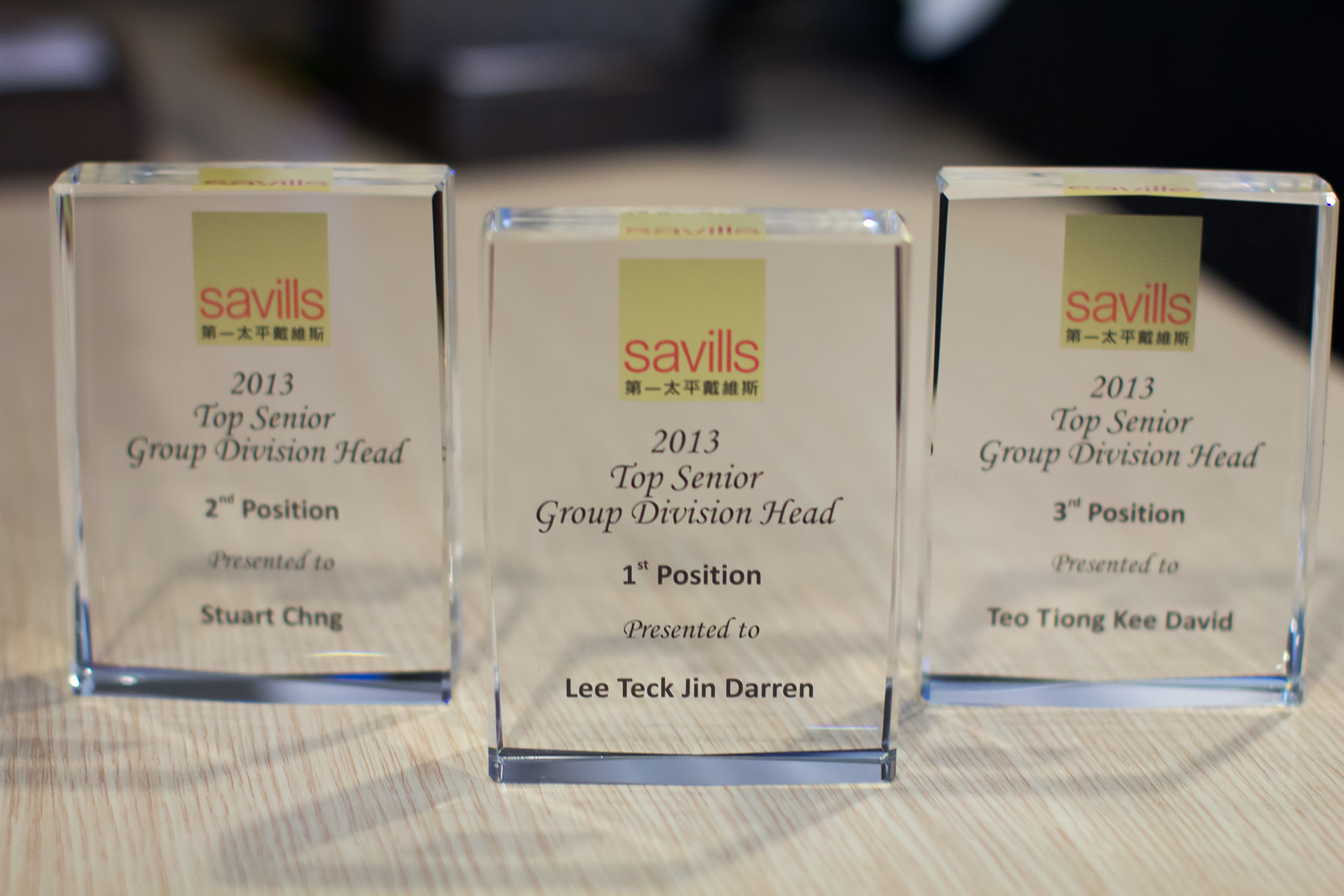The image showcases three transparent glass or lucite awards on a light-colored wooden desk. Each award is inscribed with the same yellow square logo containing red text "Savills." Below the logo, in black text, it reads "2013 Top Senior Group Division Head." The positions and names of the recipients differ among the three awards. The award in the center is for the first position, presented to "Lee Tek Jin Darren." The award on the left denotes the second position, awarded to "Stuart Chang." The award on the right is for the third position and is presented to "Theo Tiang Ki David." The background of the image is blurred, drawing focus to the awards.